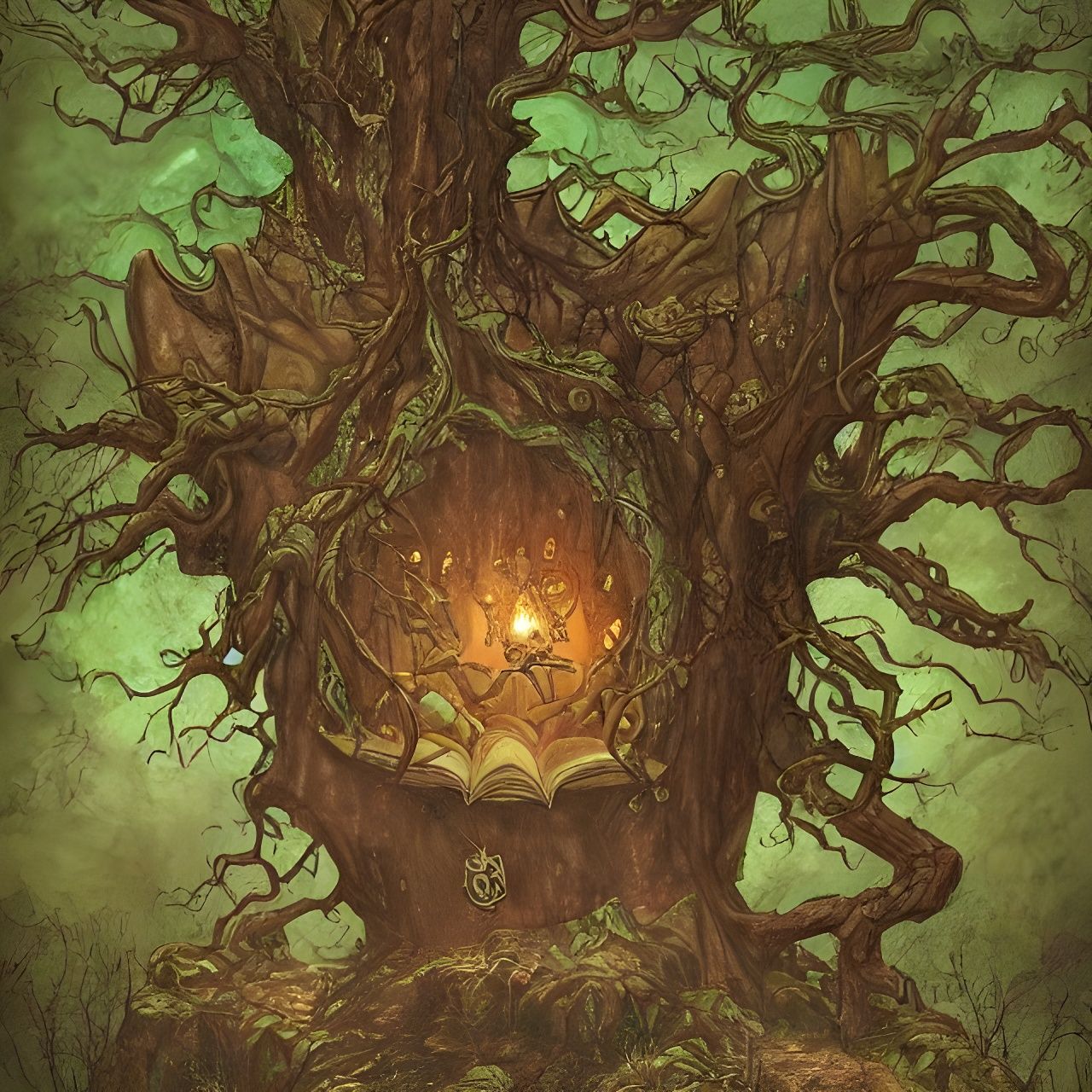This image is a digitally illustrated square depicting a fantastical and mystical tree on a solid ground or hill. The background is a mix of dark and bright greens, giving a lush, leafy, and somewhat eerie atmosphere. The tree itself is light to dark brown with numerous branches spiraling and twisting wickedly in all directions, almost resembling tentacles. The centerpiece of this unusual tree is a hollowed-out area that reveals book pages at the bottom, suggesting an open book. Radiating from within this hollow is an otherworldly glow, described as amber, yellowish gold, or flame-like, which draws immediate attention. The upper section above the hollow is covered in darker green moss and leaves, enhancing the mystical and enchanted feeling of the tree. The tree's roots extend downward into the brown and green earth, adding to the image's detailed and otherworldly charm.